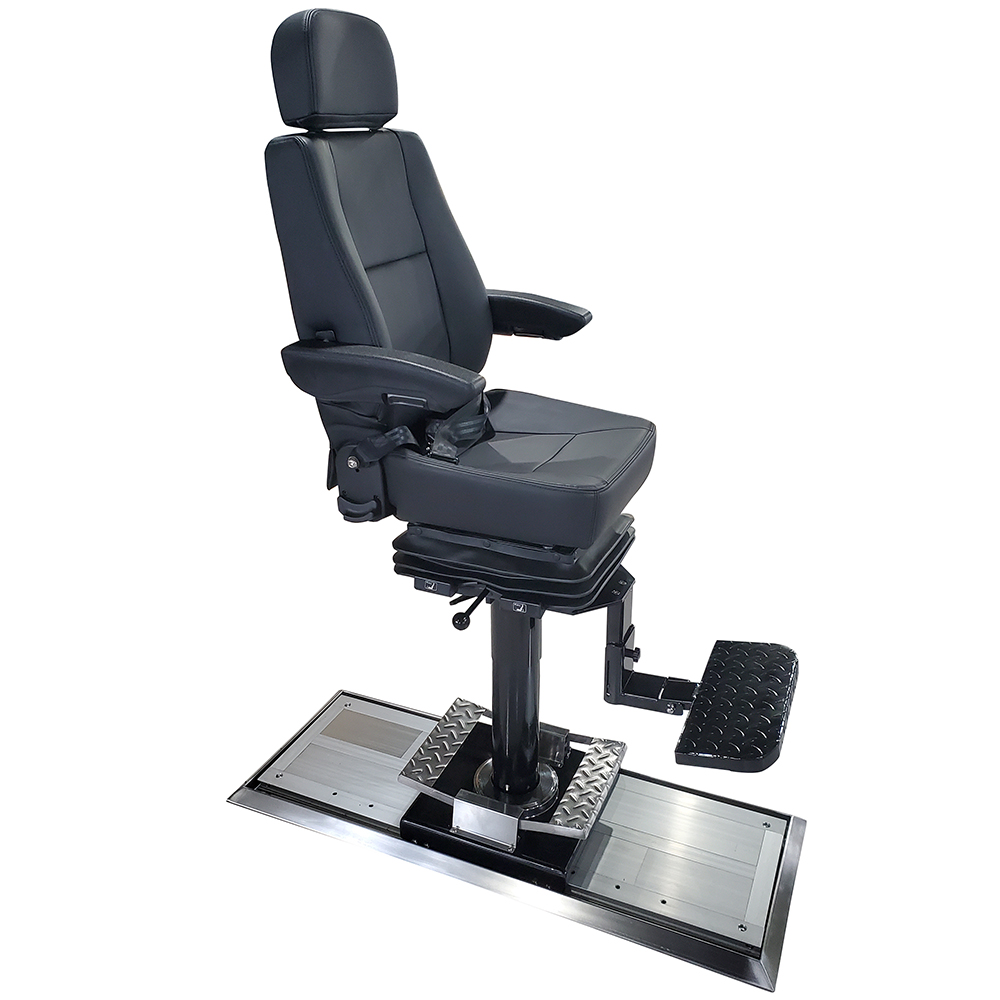The image shows a high-end, adjustable mechanical chair against a plain white background, likely a stock photo intended for a commercial product listing. The chair features a prominent metallic base mounted on a cylindrical pedestal approximately 1.5 to 2 feet tall. This base includes two chrome foot pedals for raising and lowering the seat. Rising from the base is a pole supporting the chair. The chair itself is upholstered in gray material, possibly leather, with two foldable armrests, an adjustable headrest, and a pronounced, cushioned backrest. Additionally, the seat appears roomy and well-cushioned, designed for comfort, possibly making it suitable as a fancy captain's chair. For added convenience, there is a textured metal footrest extending from the base, ensuring safe footing. The seat also includes adjustable seatbelts for security and an air cushion mechanism beneath it for further height adjustments, operated via a small handle near the bottom of the seat.